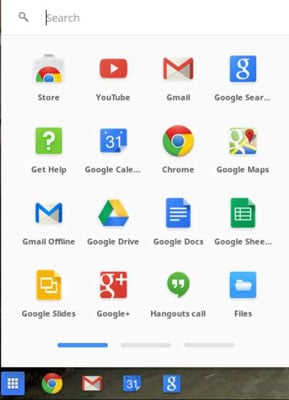The image appears to be a screenshot likely taken from a digital device, possibly a smartphone or tablet. On the left side, there is a very thin black vertical bar. At the top of the image, a white search bar spans horizontally, featuring a gray magnifying glass icon on its left side and the word "search" in gray text within it. In the search bar, a small black horizontal bar, known as the cursor, indicates where typing occurs. 

Below the search bar, there are several lines of text displaying different service names in black font. The first line lists: Store, YouTube, Gmail, Google Search. The second line includes: Githelp, Google Calendar (abbreviated as Google Cal), Chrome, Google Maps, Gmail Offline. The third line contains: Google Drive, Google Docs, Google Sheets (abbreviated as Google She). The fourth and final line enumerates: Google Slides (referred to as Google Sliders), Google Plus, Google Hangouts, and Files.

At the bottom of the image, a black horizontal bar stretches across. Within this bar are various application icons: 
- A blue square with small white squares inside
- The Chrome logo featuring red, yellow, green, and blue colors
- The Gmail logo, represented by a white envelope with a red "M"
- A blue square with a white "G"
- Several colorful icons corresponding to search functionalities.

Specifically, above YouTube, there is a red and blue logo, which is the outdated YouTube icon. The current Gmail icon is a white envelope with a red "M." The Chrome icon shows a red, yellow, green, and blue circular design. Additionally, there is a blue square with a white "G" alongside other detailed and colorful service icons.